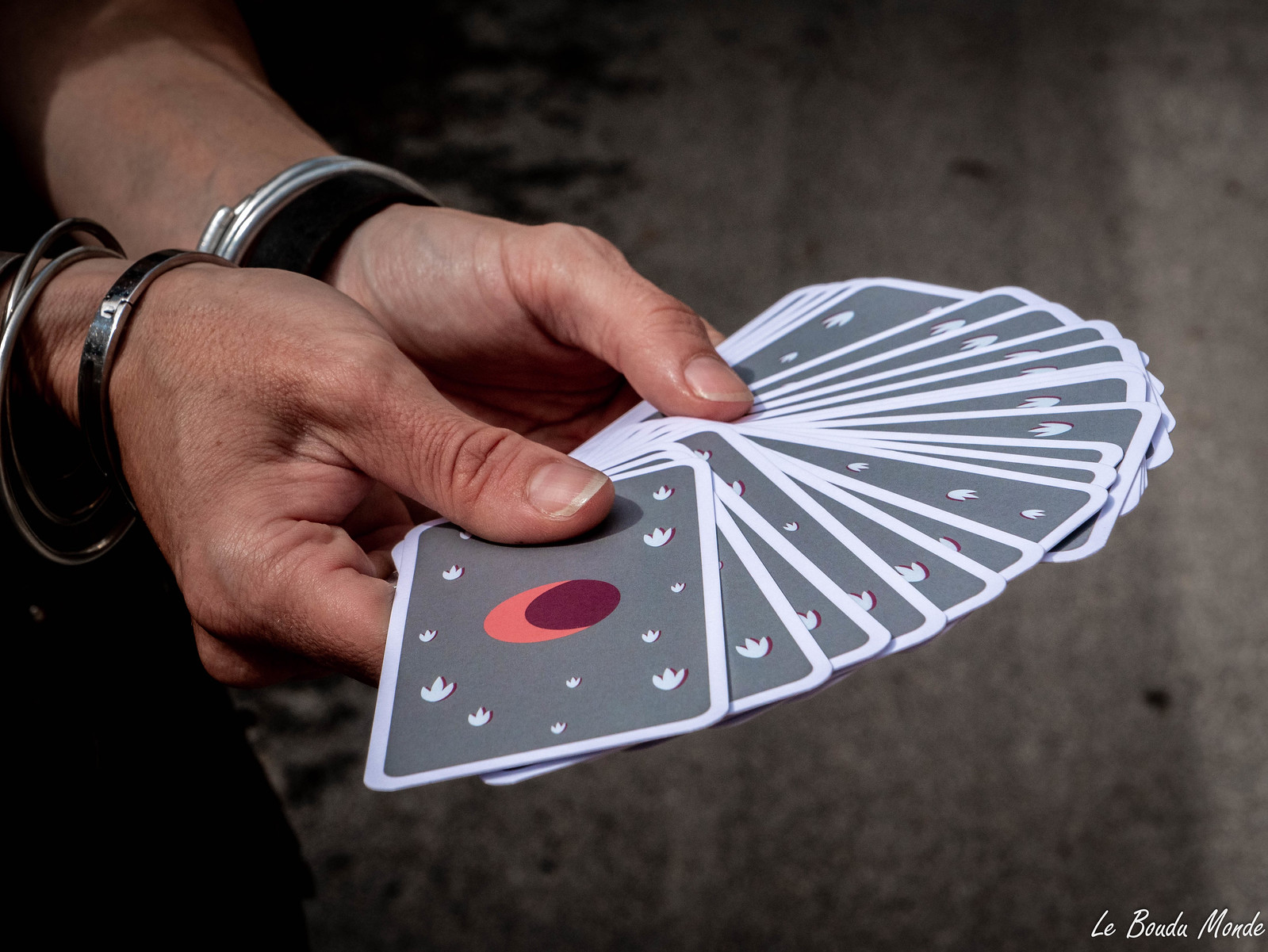In the photograph, a woman is seated on a grey-brown carpet, seemingly engrossed in tarot card reading. She holds a deck of cards delicately in her hands, which are adorned with silver bracelets—three on her right wrist and one silver with an additional black band on her left wrist. Her fingers, devoid of any nail polish, and the visible part of her forearms are intricately detailed in the image. The deck she's holding appears to be fortune-telling cards, distinguished by their grey backs featuring delicate white lotus-like designs and a striking maroon full moon with a salmon-colored crescent. The background on the left side of the photo displays large, purplish, maroonish decorations that add a mystical aura to the scene. This captivating visual, hinting at a ritual of fortune-telling, is complemented by the inscription "La Boudou Monde" in the lower right corner.